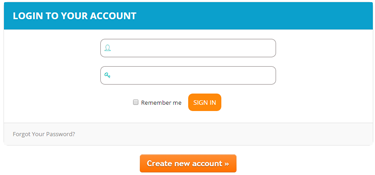This image depicts a login screen, captured either from a phone or a computer display. At the top, there is a teal-colored header with the text "Log in to your account" prominently displayed in white. Below the header, the main background area is a white rectangle.

Within this white rectangle, there are two additional smaller rectangles. The first contains an icon representing a user, while the second features a key icon, indicating fields where the user can input their username and password. Next to these fields is a checkbox labeled "Remember me."

Beneath these input fields is a prominent orange "Sign In" button. Following this, there is a gray rectangle containing the text "Forgot your password?" with a question mark, offering a recovery option.

At the bottom of the screen, a longer, orange rectangle states "Create new account," prompting users to register a new account. This section also includes two right-pointing arrows, suggesting navigation to the account creation screen.

The overall design is composed of a series of nested rectangles in teal, white, gray, and orange, creating a structured and user-friendly interface for logging in or creating a new account.